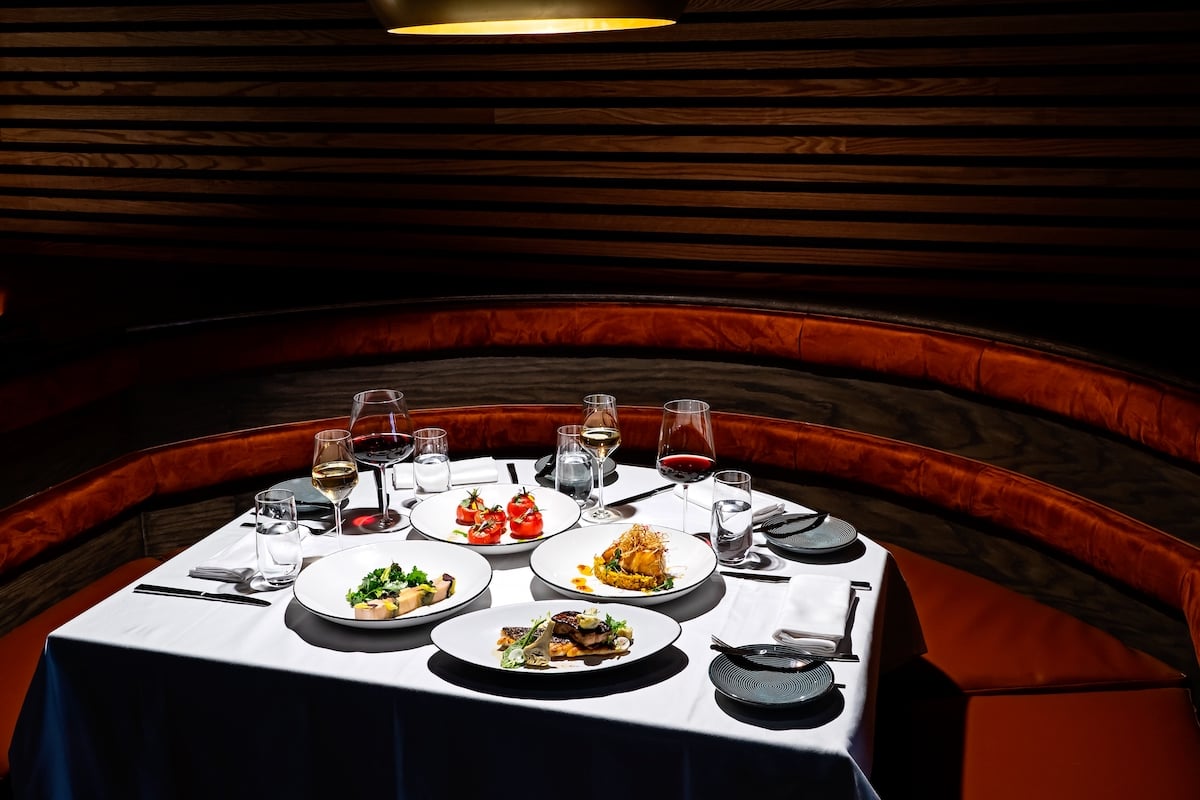The photograph showcases a sophisticated restaurant table setting. Dominating the scene is a beautifully curved wood-backed bench with rich, velvety red cushions, creating an inviting and luxurious seating arrangement. The top and bottom of the bench feature additional red velvet cushions for extra comfort. Above the table, a round, yellow lamp casts a warm glow, highlighting the elegant details of the setting against a backdrop of warm wooden slats with subtle black spacing.

In the center, a large, pristine white tablecloth covers the table, upon which gray and white plates are carefully arranged. Each place setting includes polished silverware, folded white napkins, and tall glasses of red wine alongside shorter glasses containing a golden-hued white wine and champagne. Four plates of assorted gourmet dishes are displayed: one features what looks like a steak accompanied by vegetables, another showcases bright red ingredients, possibly tomatoes, while the remaining two plates present orange and green elements, indicative of diverse and colorful culinary creations.

The ambiance, complete with a combination of textured velvet, sleek tableware, and sophisticated lighting, paints a picture of fine dining in an elegant and warm restaurant environment.